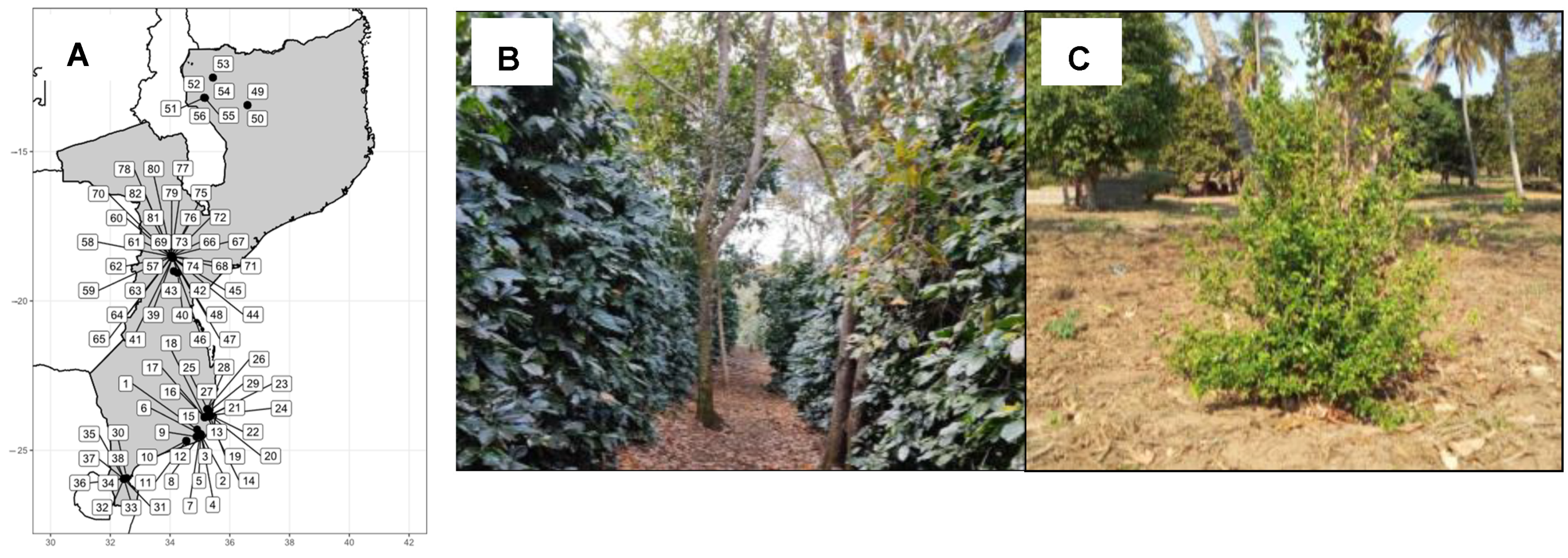This composite image consists of three labeled sections, each depicting distinct scenes. The leftmost image, labeled A, is a detailed black and white map with multiple numbered boxes connected by arrows to specific points within a shaded Y-shaped region. These numbers likely indicate notable landmarks or important locations within the mapped area. The middle image, labeled B, features a picturesque brown pathway framed by manicured hedges on either side. Amidst the hedges, two trees are visible, with their leaves hinting at spring. The pathway stretches into the background, offering glimpses of additional foliage. The rightmost image, labeled C, displays a solitary bush situated on a sparsely grass-covered plot of land. Beyond the bush, several trees, including distinctive palm trees, populate the background, leading into a small wooded area.